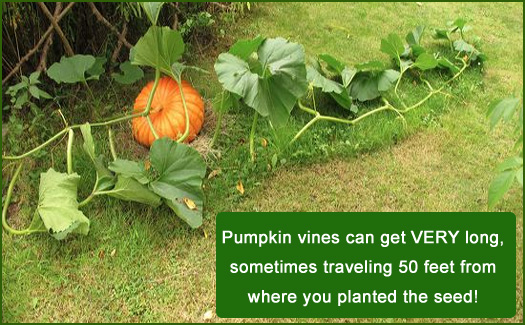The image is a portrait-mode infographic illustrating the growth of a pumpkin plant. At the center of the scene, a large, orange pumpkin is attached to a sprawling green vine, which extends across a grassy area that has been mowed around its perimeter, leaving taller grass where the vine lays. The leaves of the vine vary in size; small and sprouty near the stem and growing larger as they approach the pumpkin. The bottom right corner contains a dark green box with white text that states, "Pumpkin vines can get very long, sometimes traveling 50 feet from where you planted the seed." The top left corner features a darker brown area with dead overgrowth and stacked sticks arranged in an X-like formation, adding contrast to the vibrant greens and yellows of the grass and leaves.